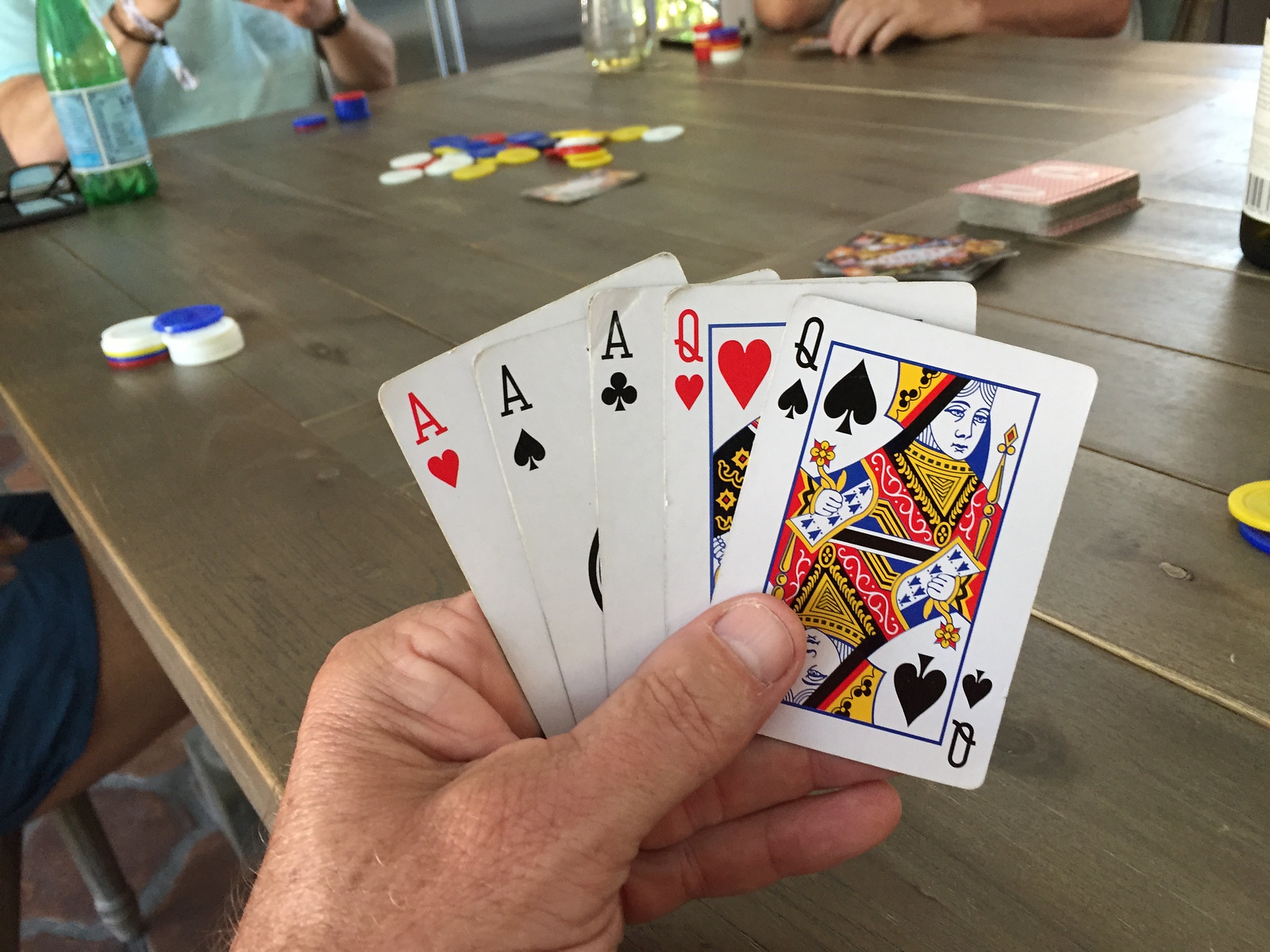In this vibrant image, a long, light brown wooden table serves as the battleground for an intense card game involving four players. At the forefront, a man's hand is prominently featured, revealing a strong hand of three aces and two queens. Beside him, a woman in shorts is partially visible, with her legs peeking into the frame. She has a mixed stack of white, blue, and red poker chips in front of her.

The table is dotted with various items adding to the lively atmosphere: a pair of glasses lays casually alongside a green bottle with a blue wrapper. At the far end, another participant in a short-sleeved blue shirt is deeply engrossed in the game. This person has a ribbon and a bracelet on their wrists, along with a watch with a brown band, and their chip stack includes blue and red chips.

Scattered around the table are a few more items: a clear glass bottle with a golden reflection, another player's hand with cards faced down, and towards the right edge, a dark-colored bottle with a white label. In the middle of the table, red-backed cards, some turned face up displaying colorful designs, are flanked by a sprawling pile of mixed poker chips in white, yellow, red, and blue – a testament to the high-stakes game unfolding.